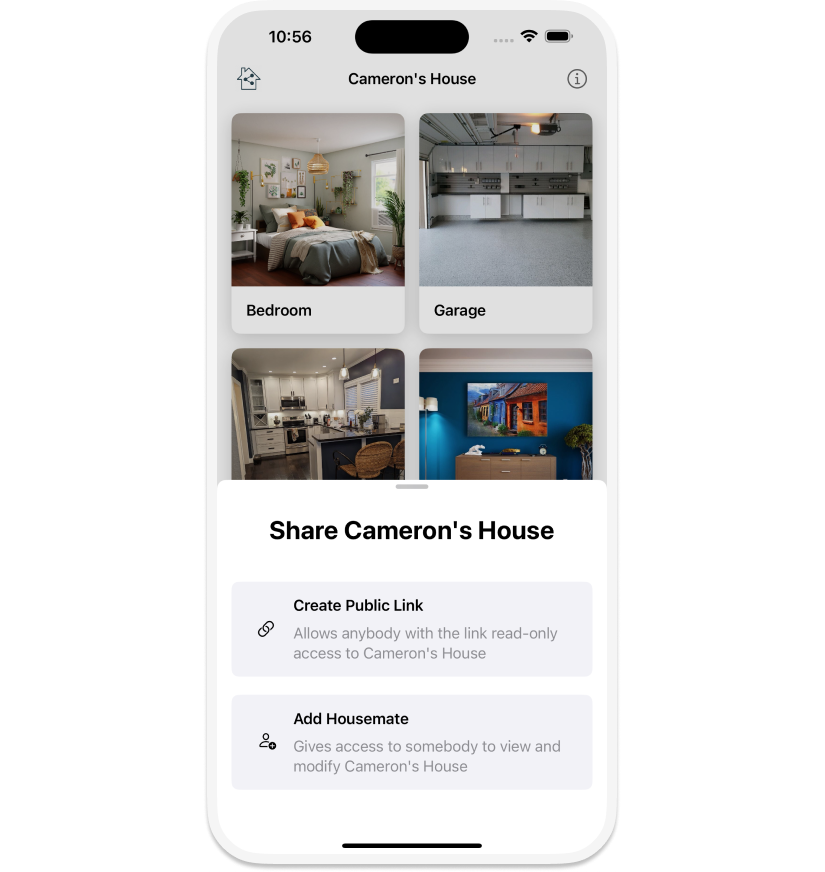The image portrays a white cell phone set against a white background. The phone displays a home screen, with the time "10:56" shown in the top left corner. To its right are icons indicating Wi-Fi connectivity, cellular signal strength, and a fully charged battery.

At the very top of the screen, in black text against the white background, the title "Cameron's house" is displayed. Below this heading, there are multiple thumbnails of photos labeled with their respective locations such as "bedroom" and "garage." Partially visible, two additional photo thumbnails are cut off from the frame.

A pull-up menu appears on the screen, featuring options in black font over a white background. The first option, "Share Cameron's house," creates a public link permitting read-only access. The second option, "Add housemate," grants someone the ability to view and modify settings within Cameron's house. These menu options are housed within horizontally oriented, gray rectangles.

At the bottom part of the screen, a black divider line runs across the middle. The visual aesthetic of the app includes a palette of white, black, gray, orange, green, brown, and blue colors. While there is no explicit mention of the application's purpose, it likely serves as a house or roommate management tool.